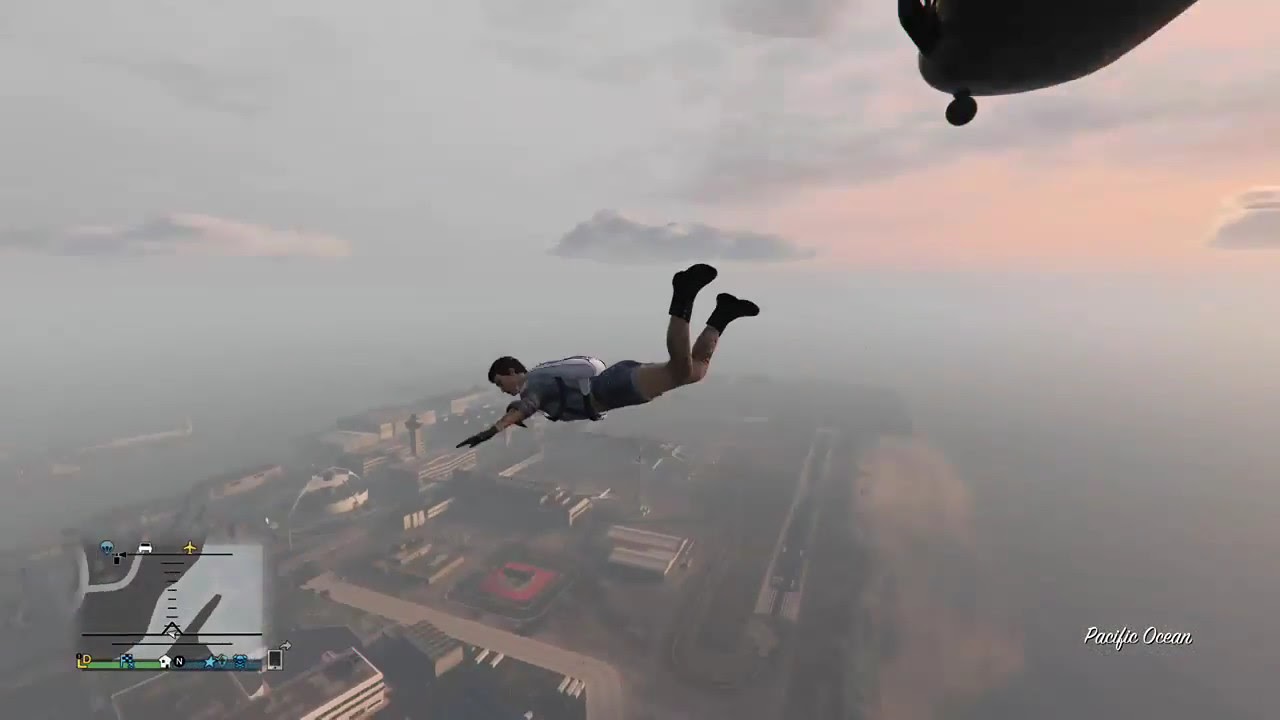In this detailed screenshot from a video game reminiscent of Grand Theft Auto, we see a Caucasian man, who appears to resemble a GI Joe character, skydiving in the center of the frame. He has short brown hair and is wearing a white shirt with the sleeves rolled up, dark gray shorts, black boots, and gloves. Positioned in a freefall with his arms outstretched and legs bent at the knees, he is descending above a mist-covered city with visible homes and buildings below. The sky is filled with a mixture of blue, gray, and dark clouds.

In the top right corner of the image, the underside of an aircraft is partially visible, indicating where the man has jumped from. The bottom left corner features an altimeter, a square instrument displaying their height above the ground. Additionally, there is a navigation map, aiding the player’s orientation. In the bottom right corner, the words "Pacific Ocean" are written in white cursive, adding to the immersive details of the scene. Overall, the combination of detailed character design, city landscape, and navigational elements highlight the dynamic and engaging visual experience of the game.